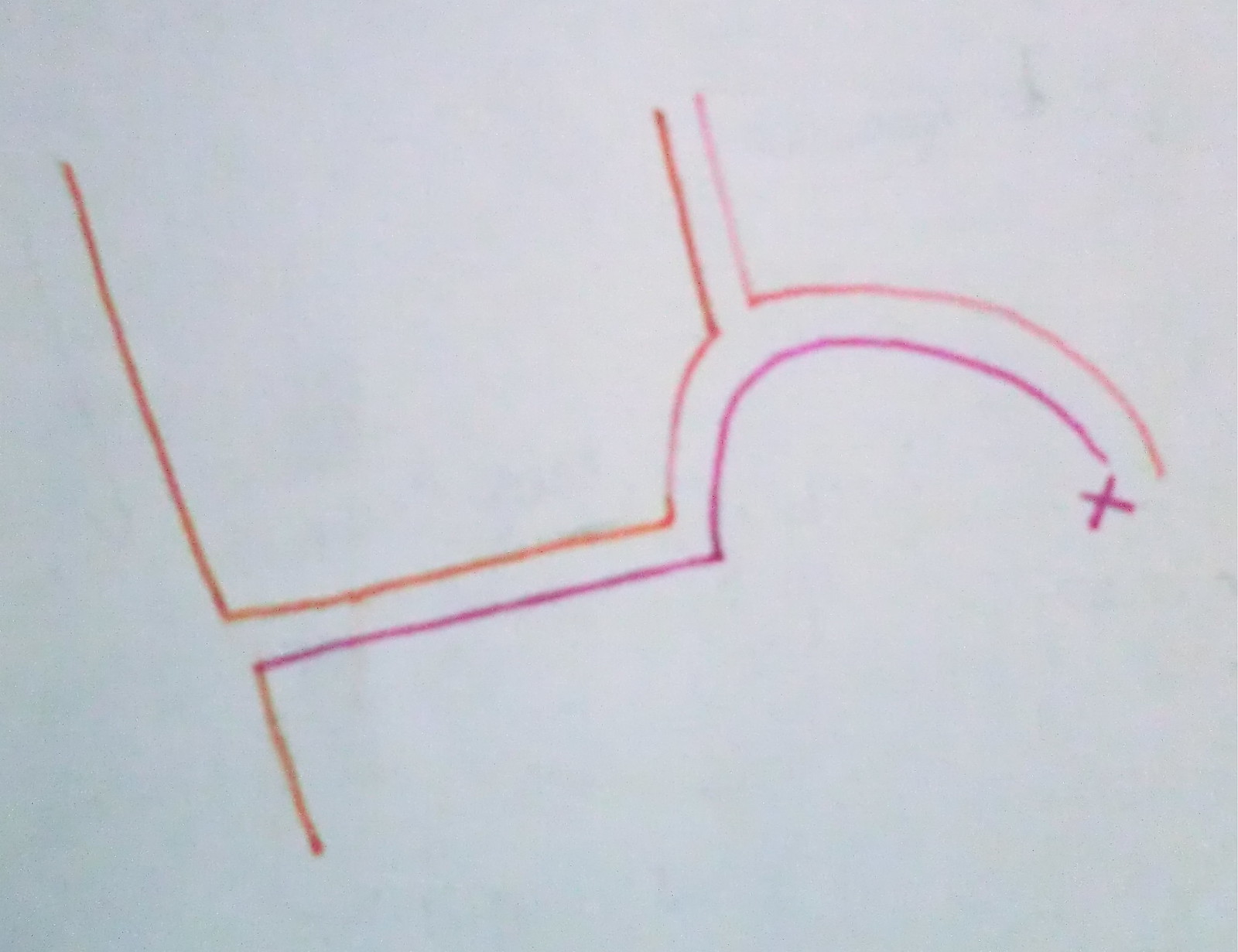The image features a white sheet of paper as its backdrop. Starting from the left, an orange line is noticeable, followed by a gap. From this gap, a yellow line begins at the bottom and scrolls upward, transitioning into a reddish-pink line that extends horizontally to the right. This reddish-pink line curves before ending at a point marked with 'NX' in the same reddish-pink color.

Descending from the top, another orange line makes its way downwards, then turns right, curving and ascending slightly. This second orange line is a slightly darker tone than the first. Adjacent to this is a line that starts as a faded pink, transitions back to orange, curves again, and extends slightly longer than the inner line, ending roughly halfway along the marked 'X'. The design composed of these colored lines remains unclear but presents a distinct and intricate pattern.